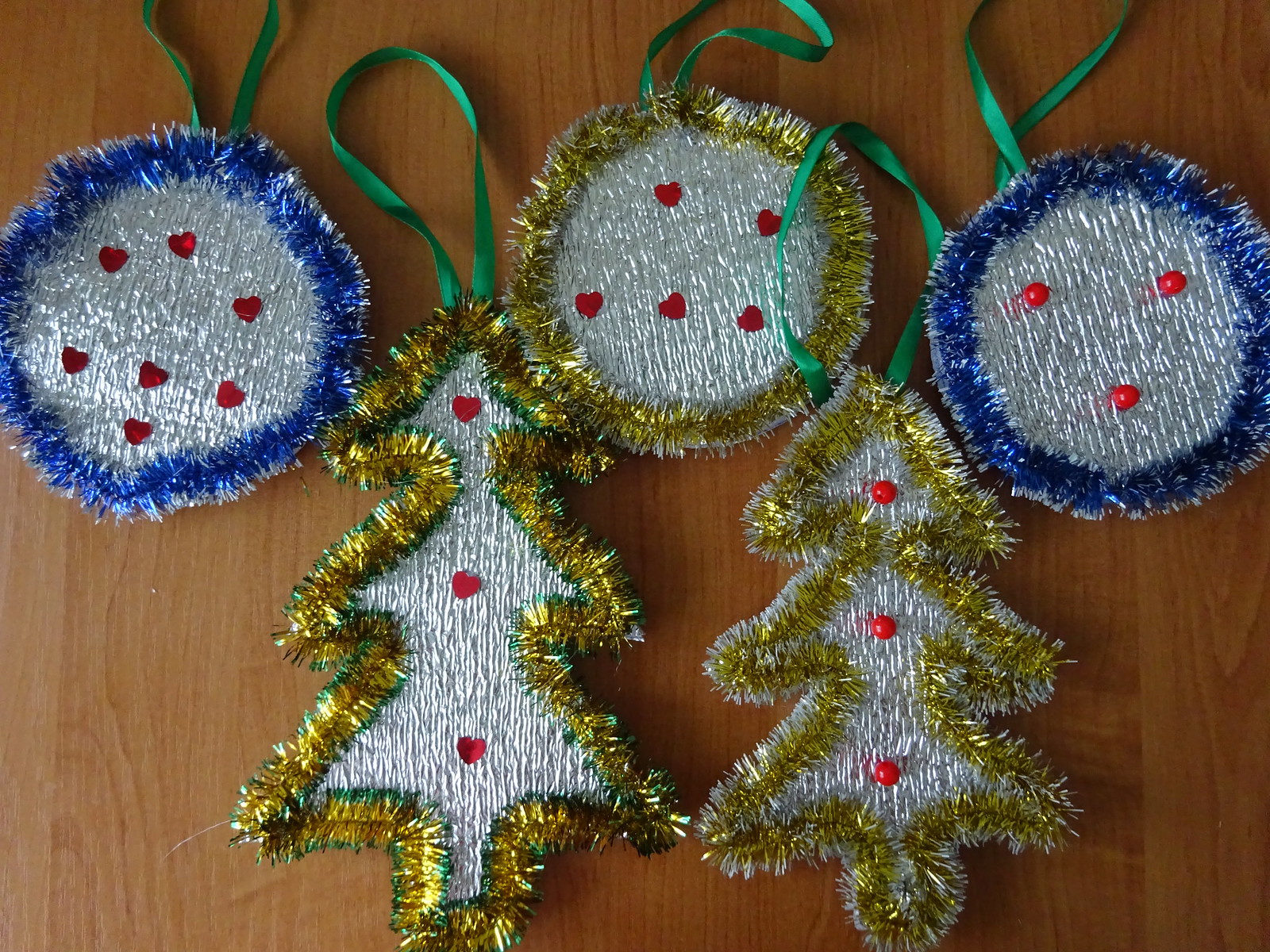This image showcases an assortment of five handmade Christmas ornaments elegantly arranged on a light brown wooden table, with the grain of the wood clearly visible. The photo is taken from a top-down perspective, emphasizing the intricate details of each ornament. At the top of the arrangement are three round ornaments, each with a silver background reminiscent of tinfoil. These are bordered by fuzzy pipe cleaners — the first on the left has a blue pipe cleaner with seven small red hearts, the second in the middle features a gold pipe cleaner with five red hearts, and the third on the right has a blue pipe cleaner with three small red balls. Below, two ornaments are shaped like Christmas trees. Both have a silver background bordered by gold pipe cleaners and are adorned with red embellishments – the first tree has three red hearts aligned in a row, while the second showcases three red balls. All five ornaments are complete with thin green ribbons attached at the top, designed for easy hanging.